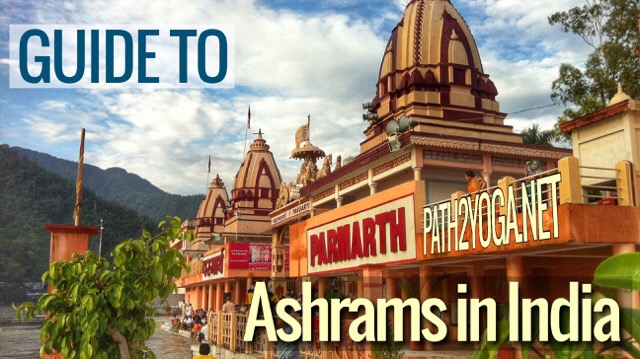The image is a promotional cover titled "Guide to Ashrams in India," with the text "Guide to" in the upper left corner and "Ashrams in India" in white at the lower right corner. It also features the website path2yoga.net. The background sky is blue with scattered clouds, adding a serene ambiance. 

On the left side of the image, there's a lush foreground with some green shrubs and a rolling hill transitioning into a mountain in the middle center background. The right side showcases multiple ashrams. The prominent ashram in the center has a large red sign that reads "Parmarth," set against a building with an ornate facade and a striking brown turret with a circular base extending skywards. This central turret is flanked by more ornate turrets and additional similar-style roofs extending along a road. 

The bottom of the image presents a mixture of green trees and architectural elements, with people seen standing on the balconies of the ashram building, all immersed in the tranquil setting. Leaves or shrubs also extend into the lower right section of the picture, adding to the lush landscape framing the scene. In the upper right corner, more trees and a building are partly visible, further enriching the detailed vista of this spiritual guide.